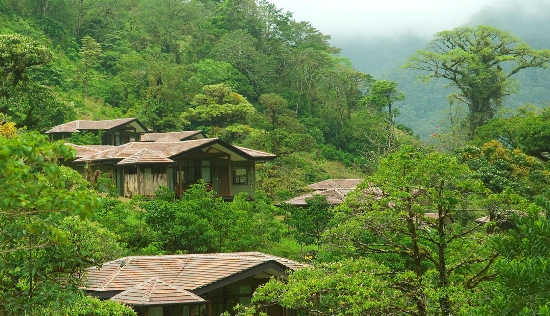This outdoor photograph captures a lush, tropical woodland scene. The dense canopy of vibrant green leaves dominates the image, especially thick and overgrown on the left side, stretching three-quarters across the frame. In the background, a fog-shrouded mountain peeks through at the top right, while patches of the sky are visible above. Nestled among the trees are several brown-roofed houses. The most prominent house, located about two inches down from the top and slightly off-center to the left, has a distinct brown wooden exterior with a darker border around its roof and windows flanking the front door. Directly to its right, another house's roof can be glimpsed, and just below this main house, a third roof barely protrudes into the bottom of the shot. Despite the image's slight blurriness, which softens the architectural details, the overall misty and elevated atmosphere gives a vivid sense of the tranquil, forested environment.